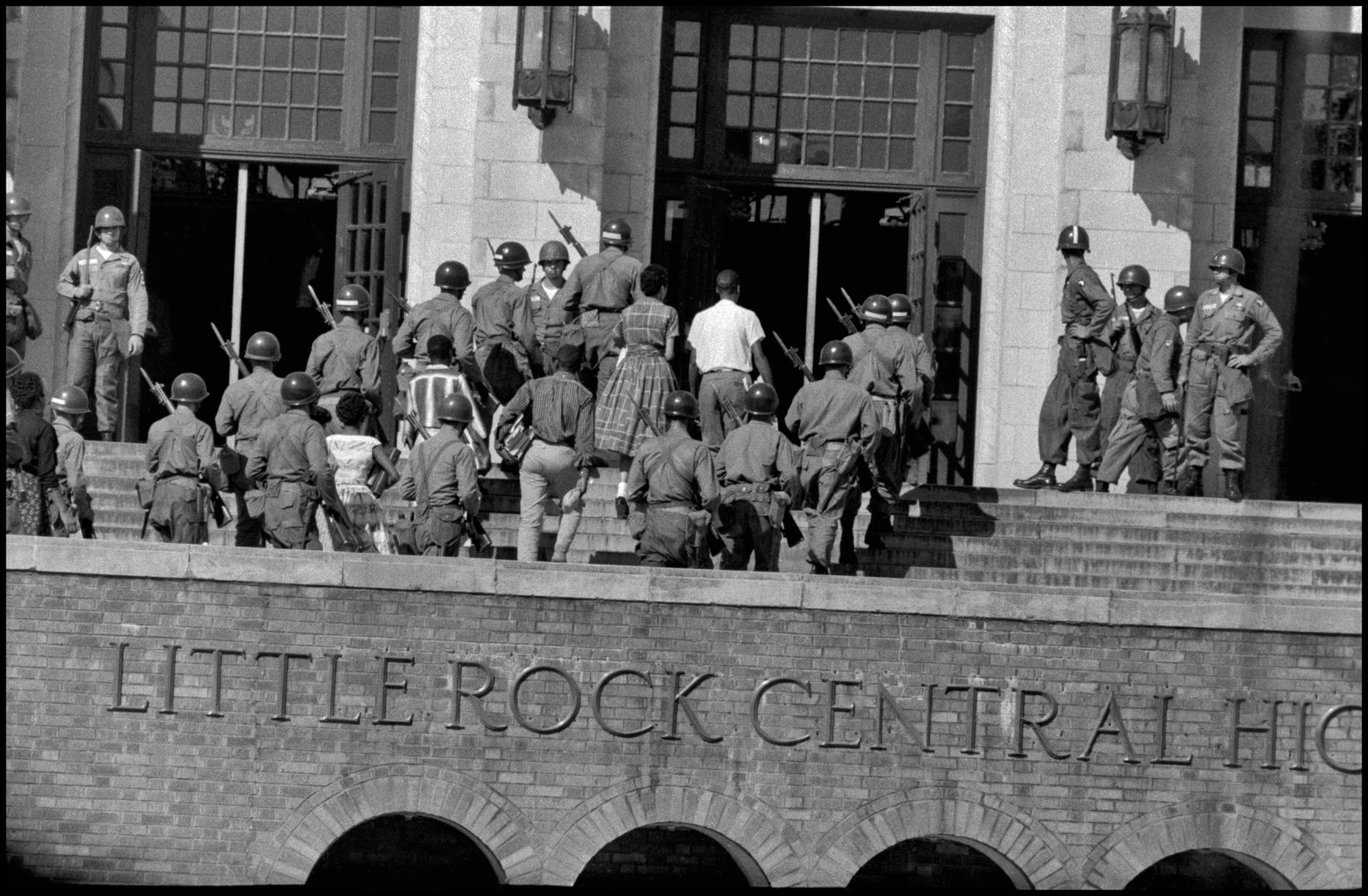This black and white photograph, likely from the 1950s or 1960s, captures a historic moment outside Little Rock Central High School. Prominently displayed is the school’s white brick façade featuring large lantern-style light fixtures and wooden double doors at the entrance. The sign "Little Rock Central" is clearly visible, though the word "High" is partially cut off at the bottom.

The photo depicts a significant event during the desegregation era, possibly the integration of the Little Rock Nine, as evidenced by the Black students entering the school. The students, some carrying books, are flanked by armed soldiers, who stand in battalion formation both at the sides of the stairs and near the doors. The soldiers wear uniforms with hard helmets and carry weapons with bayonets, clearly providing protection.

Most of the individuals in the image have their backs to the camera as they ascend the brick steps towards the school’s middle set of open doors. The students' attire reflects the fashion of the time, with boys donning shirts and jeans, and girls in full skirts and dresses, including a checkered dress and a striped outfit. This evocative photograph, showing soldiers surrounding young students entering the school, powerfully captures the tension and significance of school integration during this pivotal era in American history.